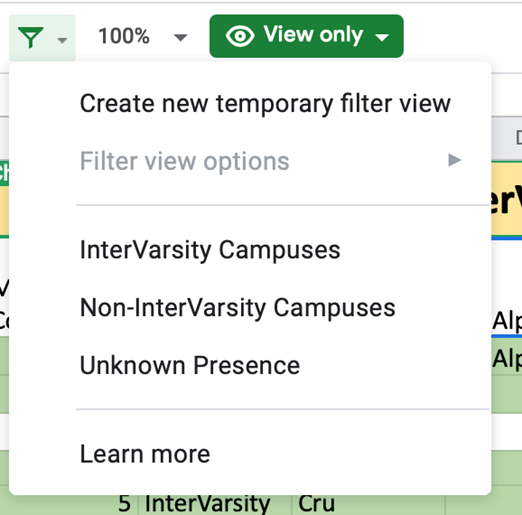A detailed screenshot of a Google Sheets spreadsheet interface is displayed. At the top, there is a magnifying glass symbol resembling a triangle with a stick vertically protruding from its bottom, followed by a downward-pointing arrow. Next to this, "100%" is shown with an adjacent downward-pointing arrow. Further along, there is an eye icon followed by the text "View only" in a green box, accompanied by another downward-pointing arrow.

In a prominent tab, a box contains the options: "Create new temporary filter view" in bold black text, with "Filter view options" in grayed-out text followed by a right-pointing arrow. Below this, categories such as "InterVarsity campuses," "Non-InterVarsity campuses," "Unknown presence," and a "Learn more" link are listed.

The background reveals a partial view of the spreadsheet, with grid lines typical of Google Sheets. Some visible text includes "Five InterVarsity CRU" and repetitive entries labeled "ALP, ALP." The majority of the spreadsheet content is obscured by the options tab. Beneath this overlay, rows and columns of cells appear, some in shades of green, and a notable yellow cell at the top containing black text. The very top of the image displays the standard Google Sheets toolbar.